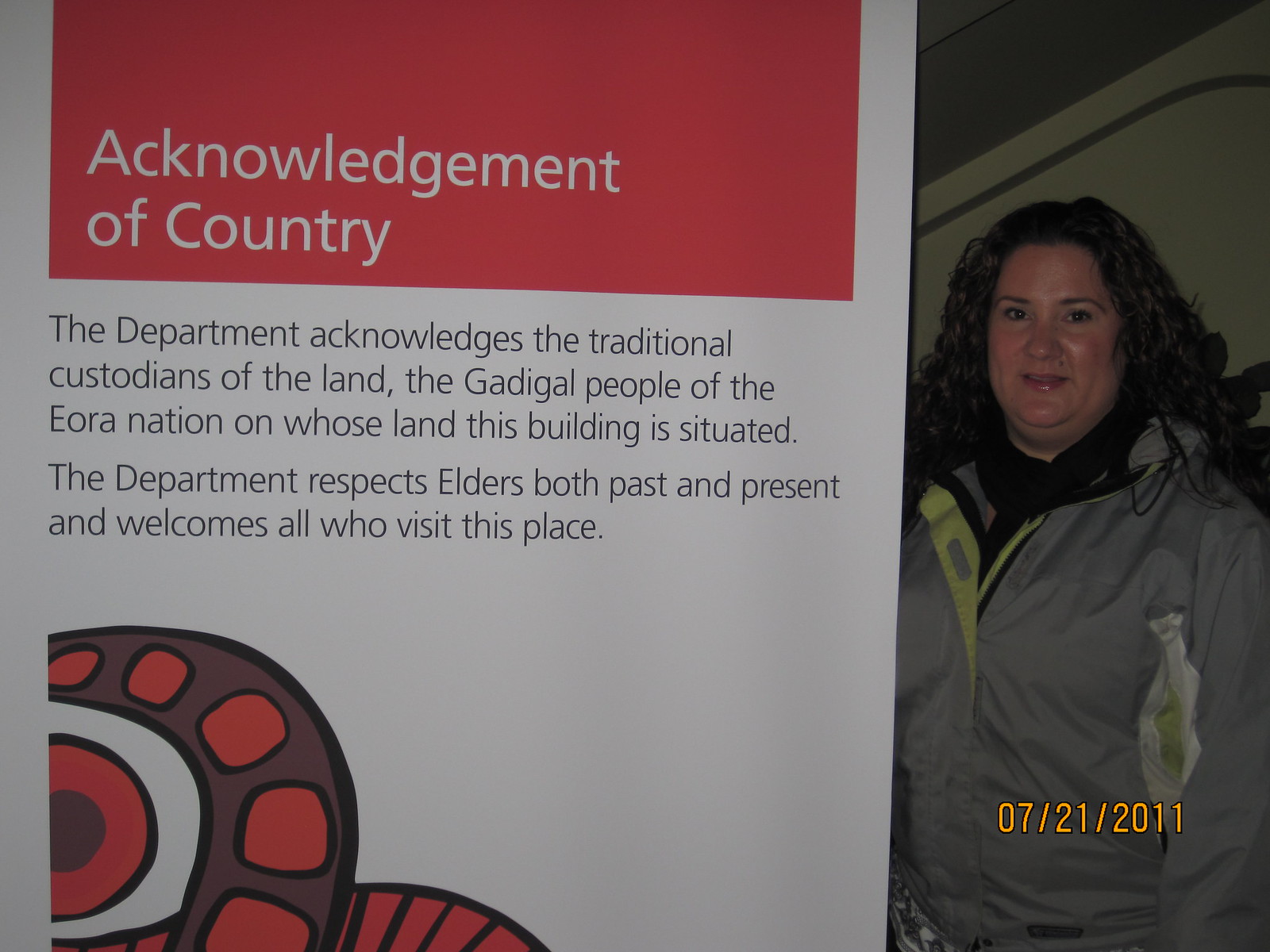This image captures a somewhat larger woman with white skin, curly brown hair, and dark brown eyes, standing on the right side of a large sign. She is wearing a gray, green, and silver jacket. Notably, she has a mole well above her right upper lip. Positioned to her left, the sign dominates the remaining space of the wide rectangular image. It features a prominent red rectangle at the top with white text that reads "Acknowledgement of Country." Below, a paragraph states, "The Department acknowledges the traditional custodians of the land, the Gadigal people of the Eora Nation, on whose land this building is situated. The Department respects elders, both past and present, and welcomes all who visit this place." At the bottom of the sign, there's a design with red and purple hues and black outlines, resembling rings around a dot. The photo is dated 07-21-2011 in orange letters above the woman.